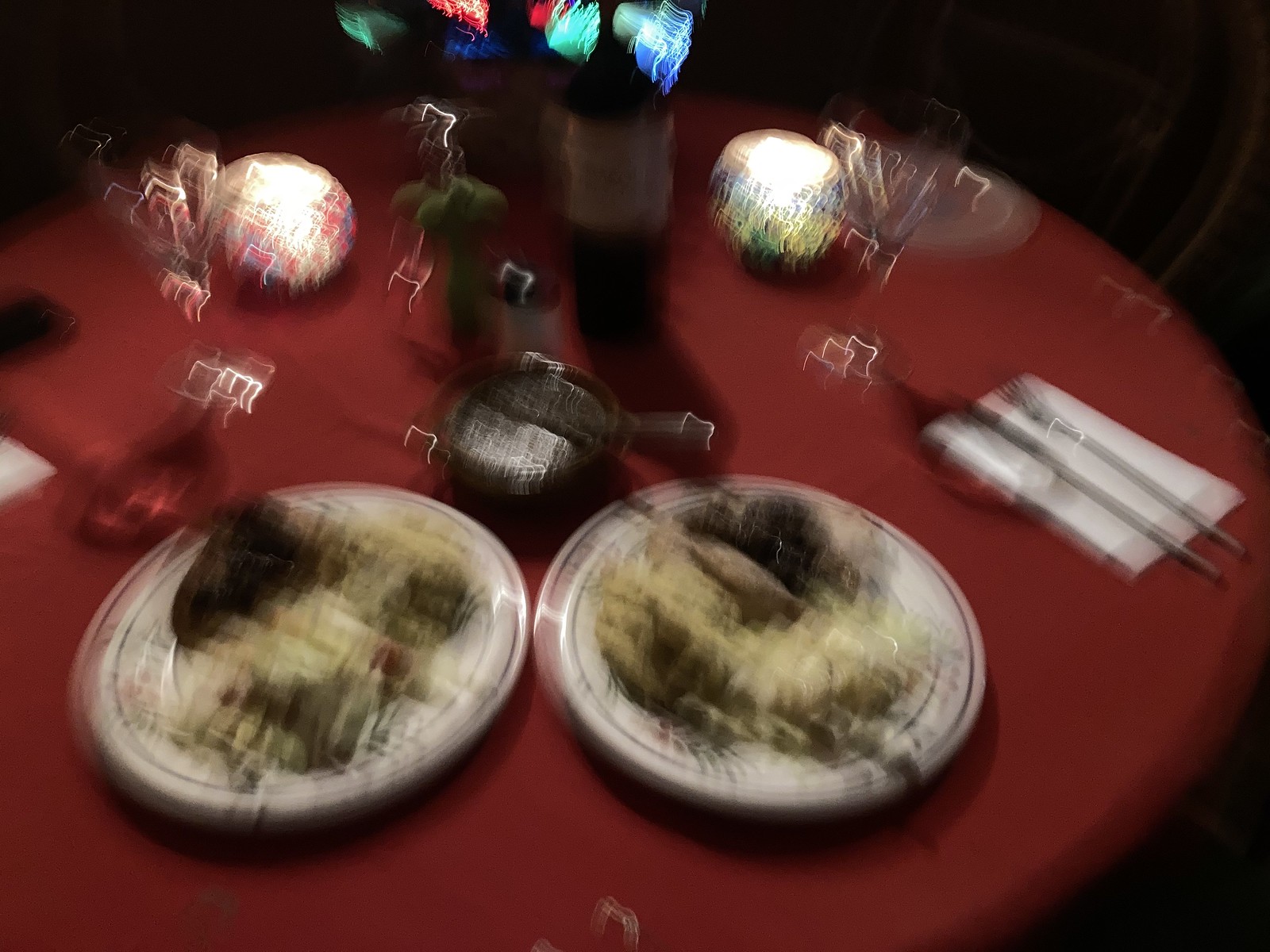This image, albeit blurry, captures a festive dinner scene. In the foreground, two white plates display identical meals, hinting at a shared experience, possibly a wedding or a celebratory event. Hovering above are some indistinct balloons, adding to the festive atmosphere. The large, round table is adorned with a rich red tablecloth, enhancing the scene's vibrancy. To the right of one of the plates lies a neatly placed fork and knife on a white napkin, suggesting a meticulously arranged setting. At the center of the table, a bottle of wine and a bowl serve as central focal points. The background remains dark, contrasting with the white, brown, and green hues of the food and the bright red tablecloth. Absent of any text or people, the image focuses solely on the dining setup, encapsulating a moment of communal celebration.